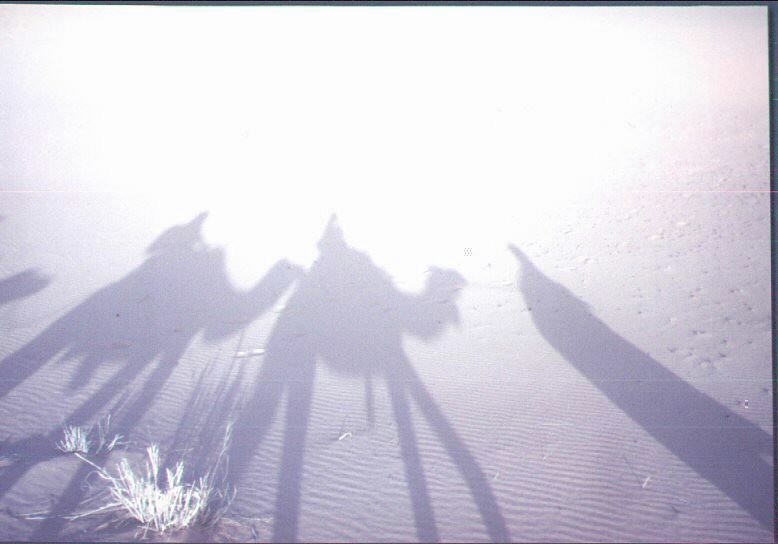This is a photograph that captures the dramatic shadows of two camels with riders and a man cast on a sandy landscape. The shadows originate from the bottom of the image, stretching towards the center, depicting elongated shapes due to the angle of the sunlight. In the scene, the two camels, with riders on their backs, progress from left to right across the frame. The riders appear to be wearing capes, magnifying their silhouettes. The legs of the camels are distinctly extended in shadow, while the shadows of the riders and the camels’ heads are clearly visible, though the back of the third camel is only suggested by a partial shadow of its head and legs further in the composition.

The sandy terrain is characterized by ripples and dimples, which add texture and depth to the photograph. Additionally, there is a conspicuous patch of dry, white grass in the bottom-left corner, contrasting against the ochre sand. The top of the image is bright and glaring, creating a stark contrast with the detailed shadows below. The photograph likely captures the perspective from the rider of the first camel, providing an intimate viewpoint of this captivating desert scene.